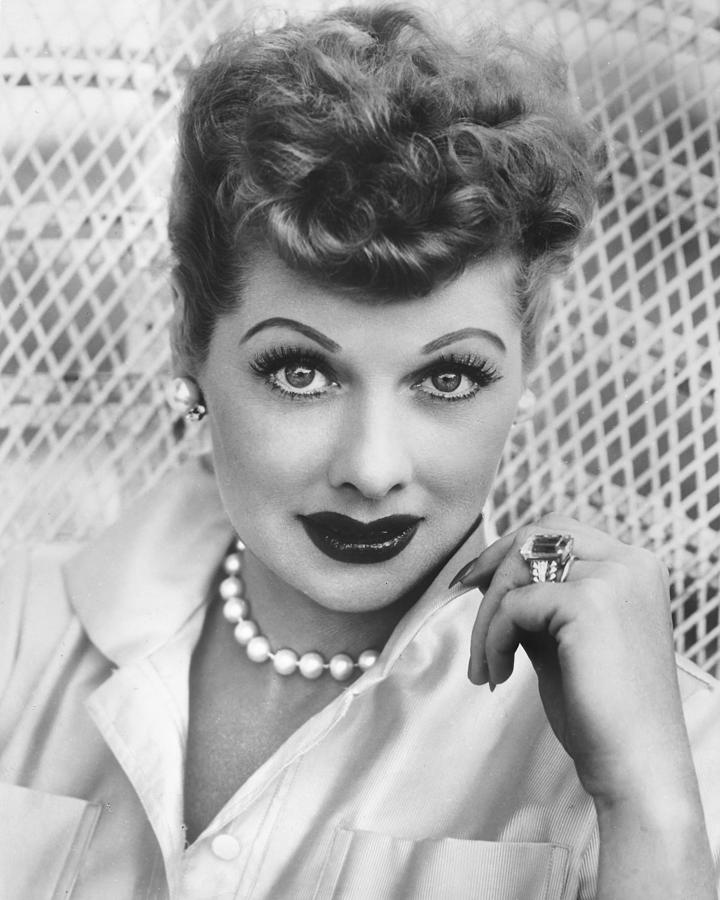This is a vintage black-and-white close-up photograph of the iconic comedian and actress, Lucille Ball. The portrait-oriented image captures her from the top of her head to slightly below her shoulders, while she sits in a white wicker fan-back outdoor patio chair. Lucille Ball, renowned for her classic roles in early television, gazes directly into the camera. Her distinctive curly red hair is elegantly styled in a bun on top of her head. She is adorned with heavy makeup, featuring false eyelashes and dark, likely red, lipstick. Large, round pearl earrings complement her tightly fitting pearl choker. Her attire includes a white satin button-up shirt with an upturned collar and two patch pockets on the chest, forming a subtle V-neck. The photograph also showcases her left arm raised near her face, fingers folded towards it, with a prominent rectangular stone ring on her ring finger. The overall style and composition reflect classic studio photography, emphasizing mid-20th-century Hollywood glamour.